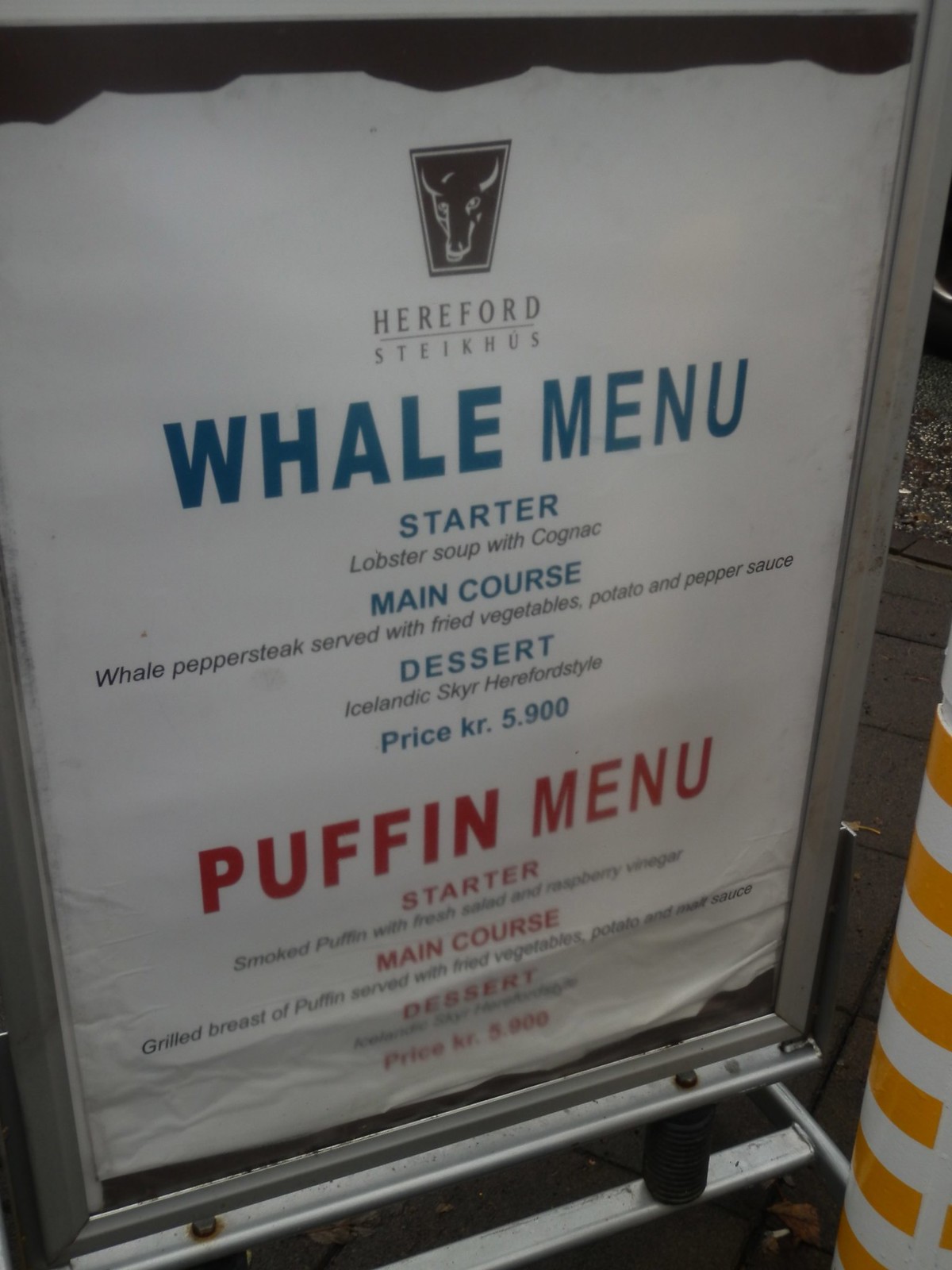The image, captured in portrait mode, features a poster menu displayed in a sign holder outside a restaurant. The sign's background is white, though slightly wrinkled towards the bottom. At the top of the poster, a distinctive steer logo is prominently displayed, under which the restaurant name, "Hereford Steinhaus," is written in black lettering. 

Just below, in larger blue lettering, the heading "Whale Menu" is presented. Following this, in smaller blue lettering, the word "Starter" is seen, with "Lobster Soup with Cognac" detailed underneath in black lettering. Further down, the menu continues with "Main Course" in the same medium-sized blue letters, describing the dish "White Pepper Steak Served with Fried Vegetables and Potato and Pepper Sauce" in black lettering.

Next, "Dessert" is highlighted in blue, though the dessert description appears blurred and partially illegible, with only "Icelandic skier" somewhat discernible. The price for this menu is listed as "KR.5.900" in black.
 
Following this section, in larger red lettering, "Puffin Menu" is introduced. Similar to the previous descriptions, it includes sections for Starter, Main Course, and Dessert, although the specific details are not included in this image.